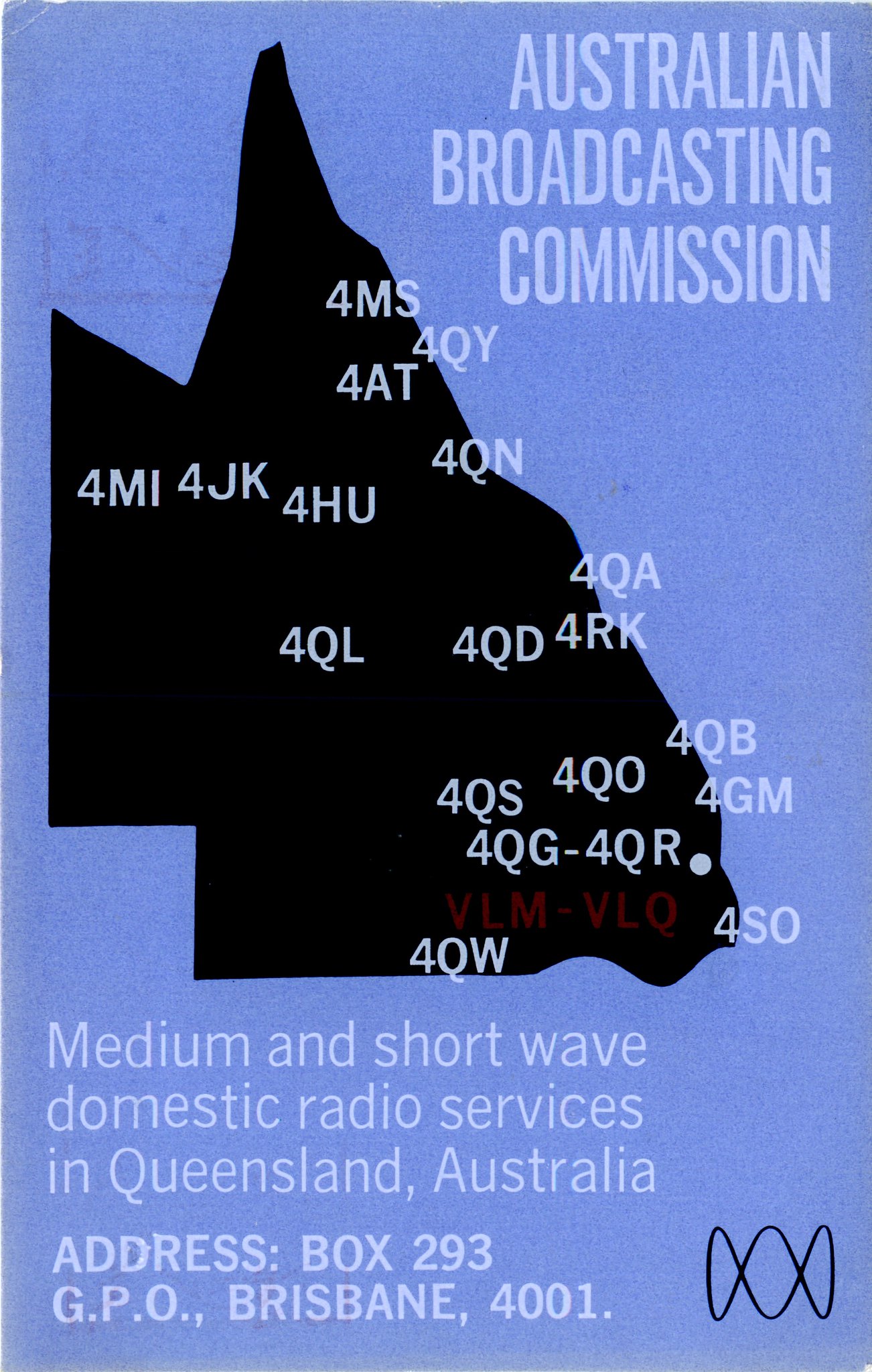The image portrays a postcard in portrait orientation, featuring a light blue background. Prominently displayed in white text on the upper right-hand corner are the words "Australian Broadcasting Commission." The centerpiece of the image is a black silhouette resembling a map, which presumably represents a section of Queensland, Australia. Scattered across this map are various white alphanumeric radio station codes such as 4MI, 4JK, 4HU, 4QL, 4QD, 4MS, 4QY, and many others, indicating different broadcasting frequencies.

Towards the bottom of the image, there is a caption in white that reads, "Medium and Shortwave Domestic Radio Services in Queensland, Australia." Below this, the address is listed as "Box 293, GPO, Brisbane, 4001." Additionally, a small black logo appears in the bottom right corner, resembling a wavelength or broadcasting signal, reinforcing the theme of radio communication.